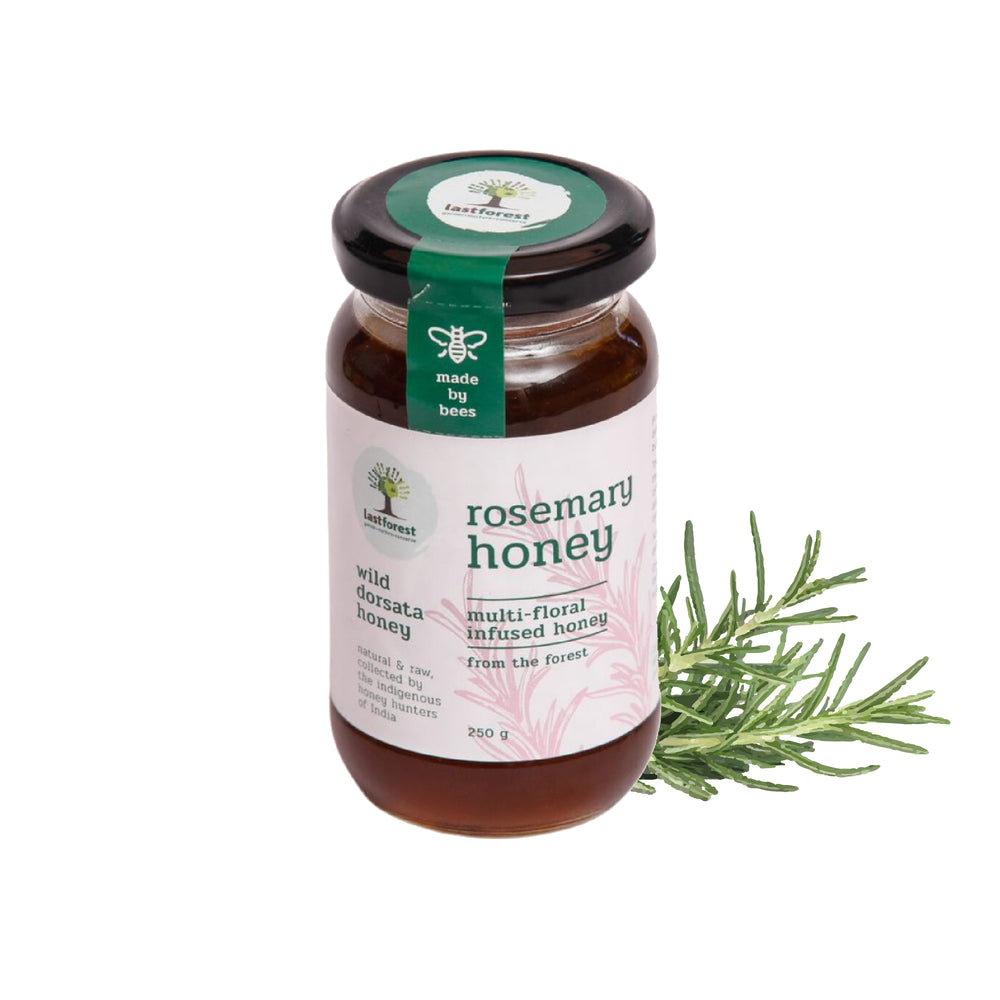This full-color photograph features a clear glass jar with a dark amber substance inside, identified as rosemary honey. The jar, capped with a black lid, has a safety sticker that bridges the jar and the lid, ensuring tamper evidence. The green label on the lid depicts a tree and includes the phrase "made by bees." The white label on the jar itself reads “rosemary honey, multi-floral infused honey from the forest” and specifies the quantity as 250 grams. Additionally, the left side of the label highlights that this is "wild Dorsada honey, natural and raw, collected by the indigenous honey hunters of India." Positioned towards the bottom right of the image is a sprig of rosemary, adding a natural touch to the presentation.